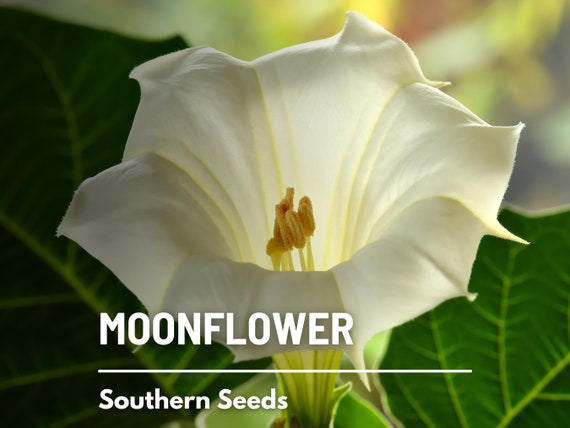This detailed outdoor photograph captures a serene and aesthetically pleasing scene with a strong emphasis on a single white moonflower, highlighted against a blurred backdrop of maroon, yellow, cream, green, and gray hues from the surrounding foliage. The flower, open and healthy, prominently displays its yellow-beige stamen in the center. To the left foreground, out-of-focus leaves add depth, while a sharply in-focus leaf on the right draws attention. At the bottom of the image, white text elegantly reads "Moonflower" in bold, followed by a thin white line, and then "Southern Seeds," giving the picture a polished, inviting look. The entire composition is softly illuminated by sunlight, suggesting it is taken during the daytime.